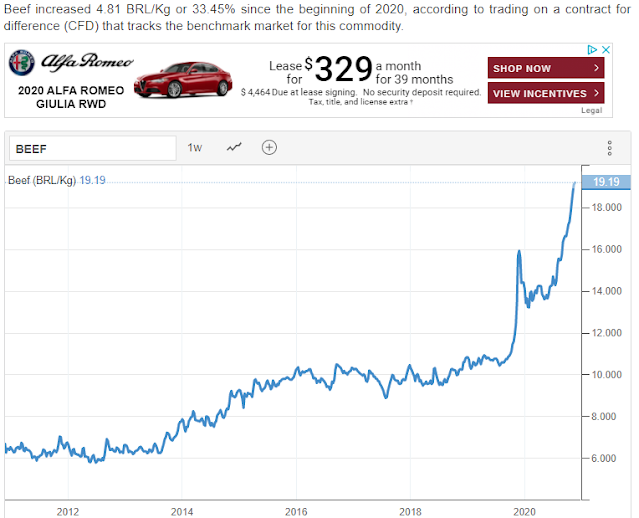The image appears to be a screenshot from a website article, featuring a graph and an advertisement. The primary background color of the image is white. There is no visible navigation bar to identify which website the article is from.

At the top, there is a block of text stating that "Beef increased by 4.81 BRL per kilogram, or 33.45 percent since the beginning of 2020, according to trading on a contract for difference (CFD) that tracks the benchmark market for this commodity."

Below this text is a rectangular landscape-style advertisement outlined in a thin gray line. The top left corner of the advert displays the Alfa Romeo badge accompanied by the text "Alfa Romeo." Below this, it reads "2020 Alfa Romeo Giulia RWD." To the right of this text is an image of a red sedan with dark windows, facing to the left. Light reflections are visible on the car's surface.

To the right of the car, the ad text reads, "Lease for $329 a month for 39 months." Immediately below, it states, "$4,464 due at lease signing. No security deposit required. Tax, title, and license extra." On the far right of the ad, there is a maroon box containing the text "Shop Now" in white with a right-pointing arrow. Below this box is another maroon box reading "View Incentives."

Below the advertisement is a graph related to the article, set against a white background with a pale gray header bar. The search tab within the header reads "BEEF" in uppercase letters. The graph displays data spanning one week, with the horizontal axis marked by years (2012, 2014, 2016, 2018, and 2020) and the vertical axis labeled with values (6, 8, 10, 12, 14, 16, 18, and 19.19).

The graph is a line graph, showing trends over time. It starts off-screen before 2012, demonstrating jagged rises and falls. Around the year 2020, the graph shows a sudden and notable upward spike towards the top of the vertical axis.